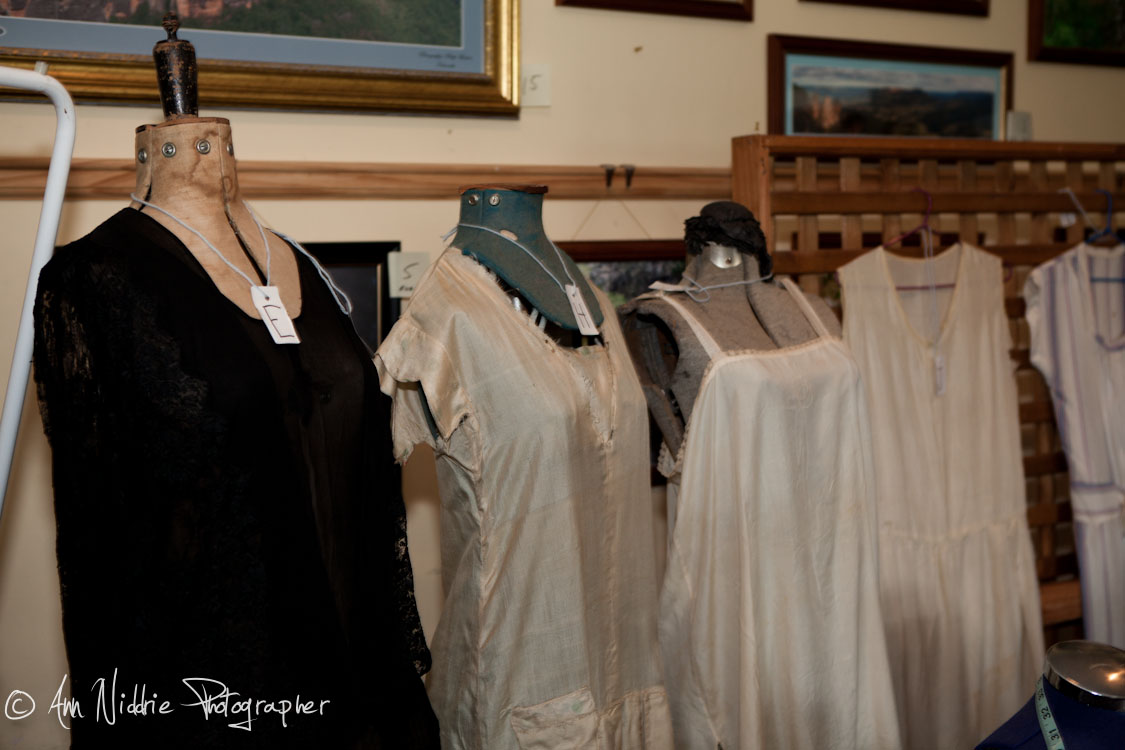This detailed photograph, credited to Anne Nidry as indicated by the white text "Anne Nidry, photographer" in the lower left corner, appears to be taken inside a vintage clothing boutique. The central focus of the image is on three headless mannequins lined up against a beige wall adorned with paintings and picture frames. Each mannequin displays different vintage dresses and has tags around their necks with black letters. The first mannequin, positioned on the left, is dressed in a black dress and has the letter "E" on its tag. The second mannequin in the middle showcases a white frock, with the tag displaying the letter "H". The third mannequin on the right is garbed in another white dress, resembling early 1900s lingerie, with its tag draped over the shoulder, making the letter indistinguishable. Additionally, to the right of the mannequins, a wooden rack holds two more light cotton or linen dresses hanging from it. The wall behind the mannequins has some brown, wood-framed art depicted in the background, completing the vintage aesthetic of this boutique store setting.